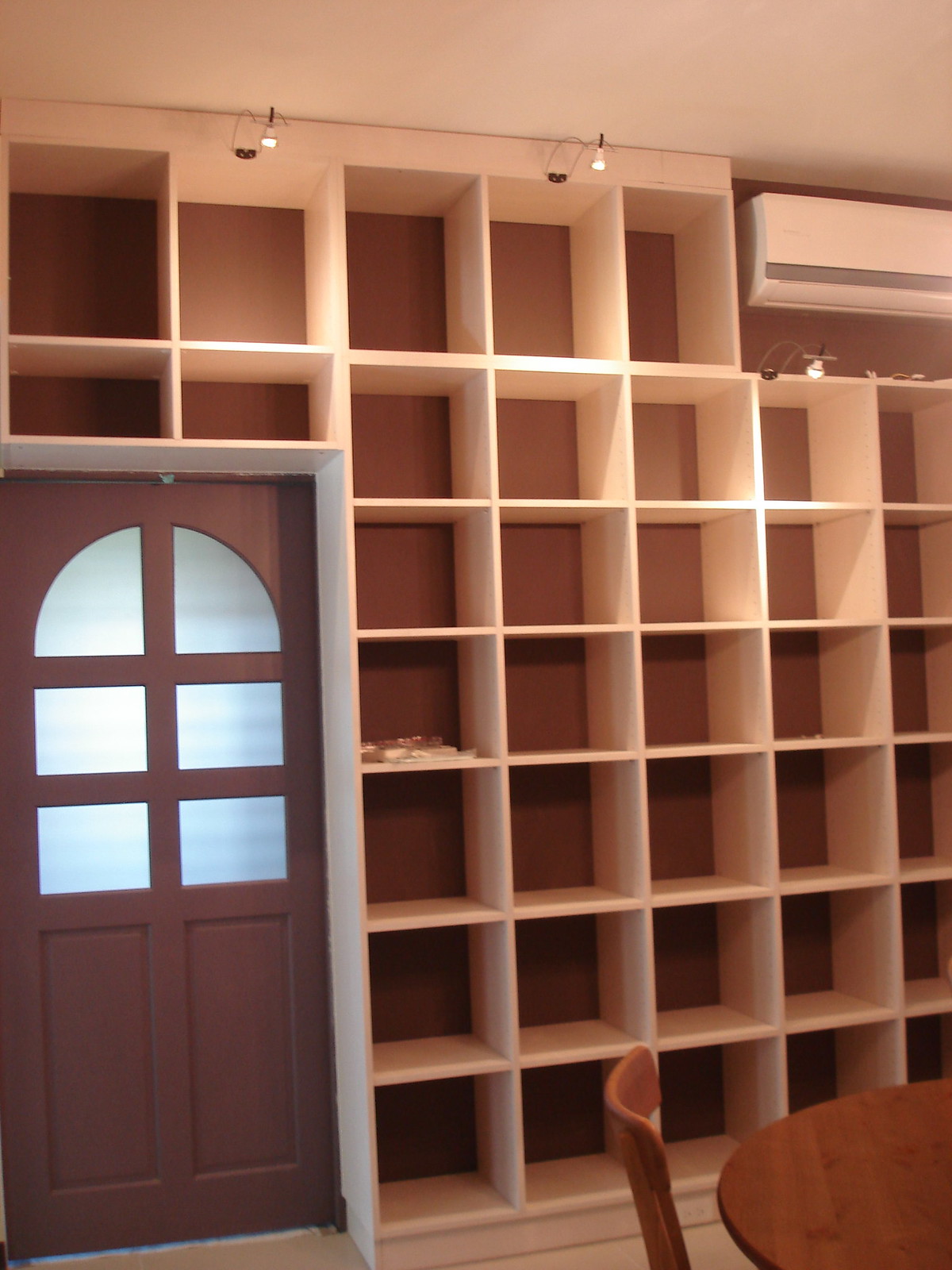This indoor color photograph showcases a quiet schoolroom or library area predominantly featuring a vast wall of white square cubbyhole shelves, extending from the ceiling to the floor. The shelving unit is composed of at least six columns, each with a minimum of five cubes, and occupies the entire wall space to the right of a distinctive dark brown wooden door. The door, situated on the left side of the image, features a cathedral-style window with six panes of glass, the top two panes forming an arch shape, with the windows occupying the upper half of the door. Above the cubbyholes on the tan ceiling, a series of small, curved pipe-mounted lights, each ending in a tiny lightbulb, provide illumination by casting light back onto the shelves. There is also an induction air cleaner or air conditioning unit mounted high on the upper right corner of the wall, beneath which another similar light fixture is visible. The interior is minimally furnished, with the lower right corner of the image showing part of a round wooden table and the back of a wooden chair in profile. Notably, the cubbyholes are primarily empty, except for one cubby near the door's midpoint containing a small stack, possibly books or mail, adding a subtle point of interest to the otherwise bare shelves.